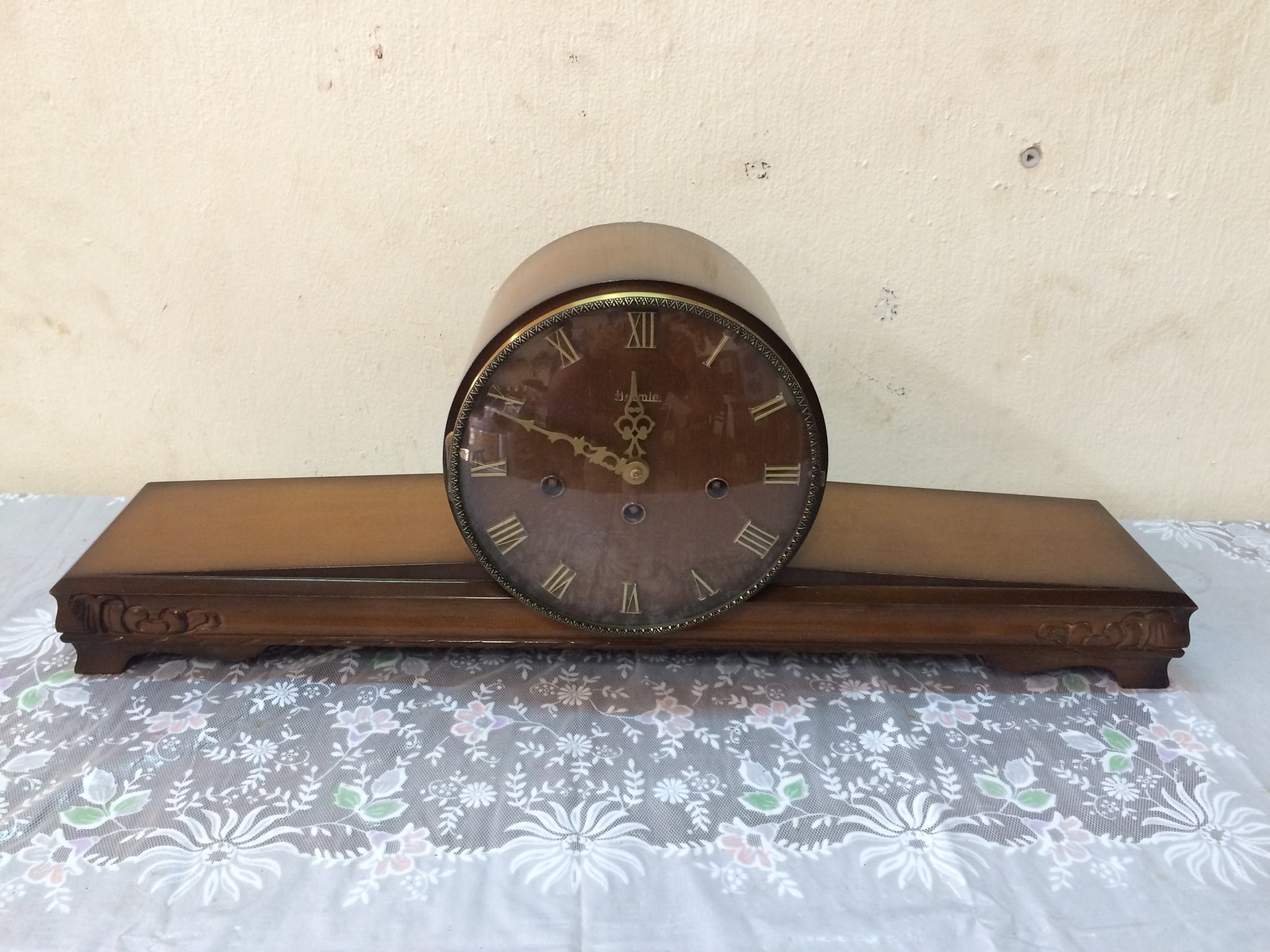This image captures an antique-style, cylindrical clock centered on a thin, dark wood slab that spans nearly the entire width of the rectangular frame. The clock features a dark burgundy red face adorned with gold Roman numerals, indicating the time is 11:50. At the bottom of the clock face, there are three small circular elements. The entire assembly rests atop a patterned tablecloth that is decorated with floral and growth motifs in shades of white, gray, and possibly blue. The background is a cream-colored wall with an eggshell appearance, showing signs of dirt or discoloration.